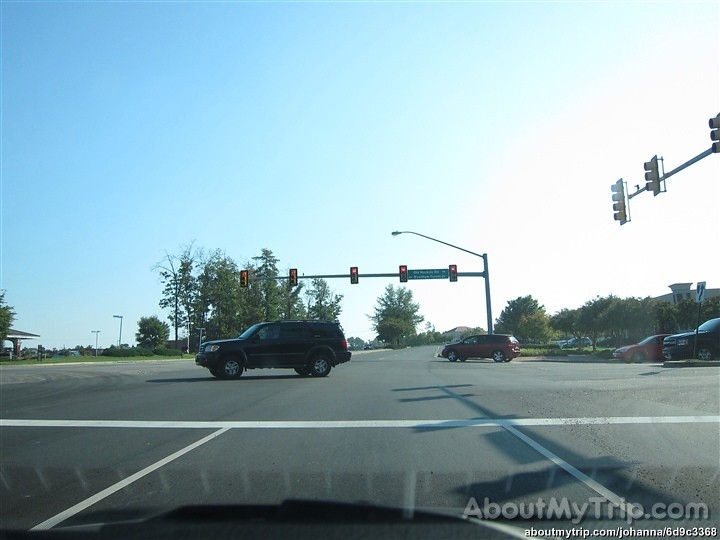This photo, captured from a dashcam, depicts a bustling intersection on a clear, blue-skied day. The dark gray asphalt street is marked with white traffic lines. At the bottom right corner of the image, a tall shadow is cast from street signs or lights above the frame. In the forefront, several vehicles navigate the intersection; a black SUV turns left, while a red SUV turns right. To the right, two cars remain stopped. The intersection's traffic signal displays a red light. Surrounding the intersection, patches of green grass and tall, leafy green trees complement a backdrop of buildings and streetlights. Prominently visible, a large streetlight with a metallic arm extends outward, supporting five sets of street lights. At the bottom right corner, the text "aboutmytrip.com/Johanna/6d9c3368" is displayed, marking the photo's origin.